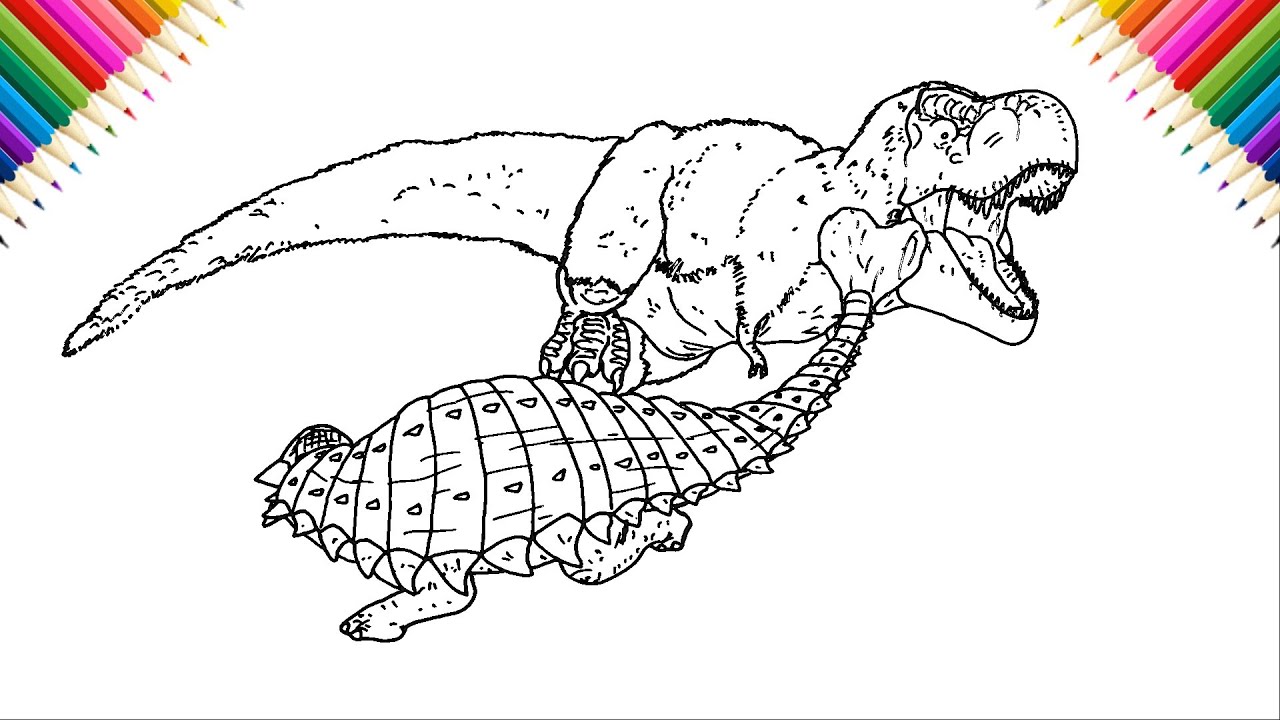A detailed black-and-white pencil sketch depicts a dramatic scene of a T-Rex attacking another dinosaur that resembles a heavily armored, turtle-like creature. The T-Rex is shown in profile with its mouth open, poised to strike. The smaller dinosaur, positioned in the foreground, appears to be using its tail, which is flipper-like and possibly armored, to fend off the attacking T-Rex. The illustration captures a moment of intense action, with the smaller dinosaur seemingly trying to use its defensive features to ward off the threat. Surrounding the image are brightly colored pencils arranged in both the upper left and right corners, pointing towards the center. These pencils include shades of lime green, dark green, blue, purple, red, light purple, orange, coral, and yellow. This arrangement suggests that the sketch might be intended for a coloring book or to encourage coloring activities. The scene, dynamic and charged with energy, contrasts sharply with the vibrant potential colors provided by the pencils, inviting viewers to bring the battle to life with their hues.